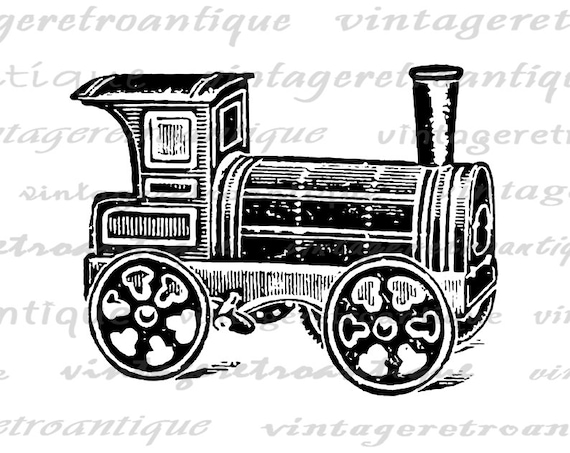This is a black-and-white drawing of a vintage child's train engine, depicted in a square image with a white background. The train engine, reminiscent of models from the 1920s or 1930s, features a visible smokestack in the front. Its little cabin at the back includes a window on the front and another on the side. The wheels are detailed with a white rim and black interior. The image lacks a definitive border, blending seamlessly into the white of the screen. Overlaid on the drawing is a blue, repetitive watermark that's difficult to read, but suggests the phrases "Vintage Antiques" and "Vintage Retro."